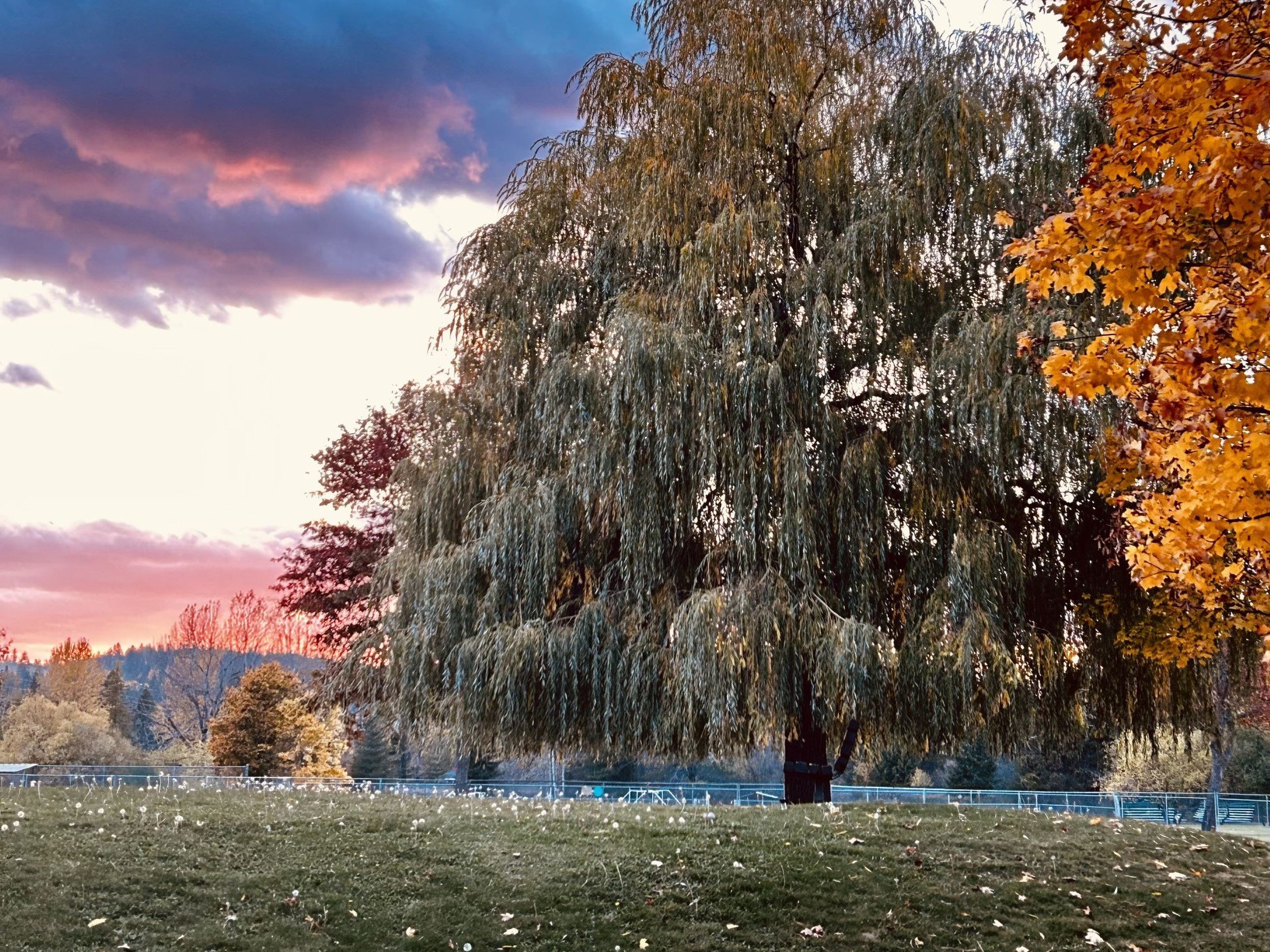This photograph captures a serene outdoor scene, likely in a park or open field during early fall at sunset. The top left of the image features a light gray sky with dark blue and light pink clouds, illuminated by the setting sun, giving hints of dull yellow and red hues. The bottom portion of the image showcases a vast expanse of grass with scattered autumn leaves. Dominating the scene is a large tree, possibly a weeping willow, with long, overhanging green leaves. To its right stands a brightly colored tree, likely an oak, with vivid yellow foliage. Smaller trees and rolling hills form the background, hinting at a peaceful landscape. In the bottom right of the image, a couple of park benches sit near a blue fence, suggesting it is a public park. The presence of a pathway, partially obscured by the trees, and some scattered dandelions add to the idyllic, tranquil atmosphere of the scene.